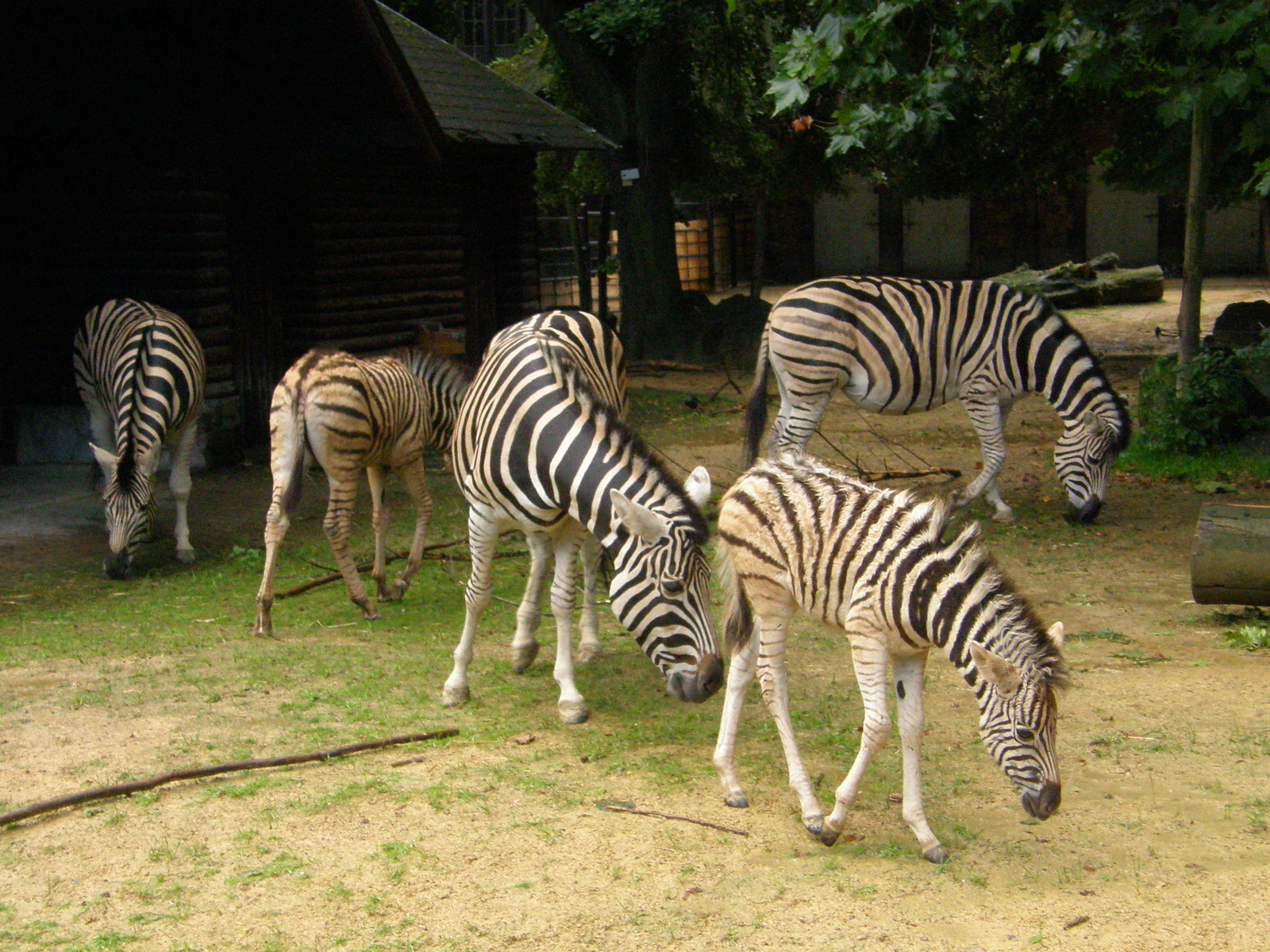In this horizontal rectangular photograph, five zebras with unique black, white, and tan markings are scattered on a slightly grassy knoll. Each zebra's head is down, appearing to search for food among the patchy grass and soil mixed with small weeds. The first zebra, located toward the lower right corner of the image, is smaller and faces the same direction. Directly behind it, a larger zebra with notably darker stripes also has its head lowered. To the left is another smaller zebra whose head is obscured by the large zebra’s body, showing only its black feet and backside. Further left, close to the left edge, a larger zebra with very dark stripes stands, its head down and facing forward. The fifth zebra is placed about two-thirds across the image and one-third down, visible in profile and facing the right-hand edge with its fluffy tail prominent.

Behind the zebras, a log cabin building stands with what looks like a lit window, adjacent to a fence and another wooden structure with three white doors. Scattered across the field are fallen tree trunks and several tree limbs, including a large stick and branches that the zebras appear to be exploring. A deciduous tree and other trees populate the background, while a large round tube and what might be part of a knocked-over pail are visible on the right side. The overall scene suggests a zoo enclosure, with the zebras peacefully grazing amid a mixture of natural and man-made elements.